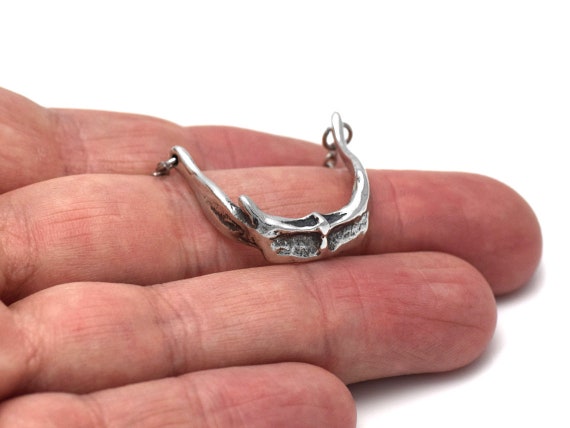The image features a person's hand extended flat, emerging from the left side of the frame against a blank, white background. The hand prominently displays a silver pendant, positioned on the middle finger. The intricate pendant resembles monstrous teeth and appears to have a somewhat ornate design at the front. Surrounding it are the soft hues of beige, gray, black, and white, contributing to the overall simplicity and focus of the picture. The pendant seems slightly cut off in the back, where subtle clipping can be observed. The scene provides no additional context or text, emphasizing the hand and the striking silver pendant it holds.